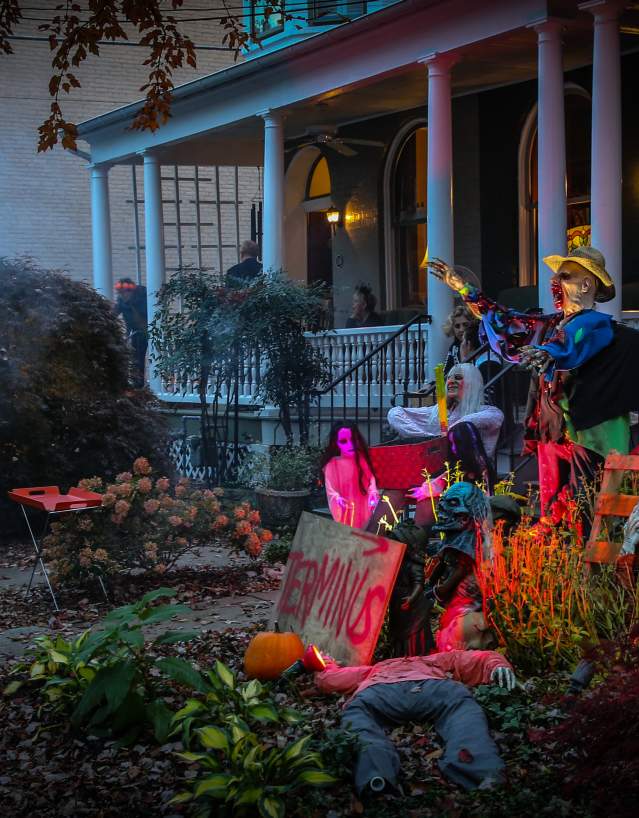This image showcases a large, gray house decorated extensively for Halloween. The house features a wide front porch bordered by white columns and a white guardrail. On the porch, several people can be seen sitting amid the spooky décor. The house is adorned with various Halloween decorations, including a sign that reads "Terminus" in red lighting. Prominent among the eerie decorations is a figure resembling Freddy Krueger, wearing a farmer's hat and a blue-and-green robe, with blood around its mouth. Below this figure is a demon-like crypt keeper.

The front yard is filled with more Halloween decorations, including an orange pumpkin, brown dried leaves scattered across the gray sidewalk, and what appears to be a stuffed figure lying flat on the ground. There's also a red tray to the left of the walkway and tall plants around the premises. A small white fence encloses the porch area, and a power line can be seen overhead. The overall ambiance is dark, adding to the spooky atmosphere of the scene.